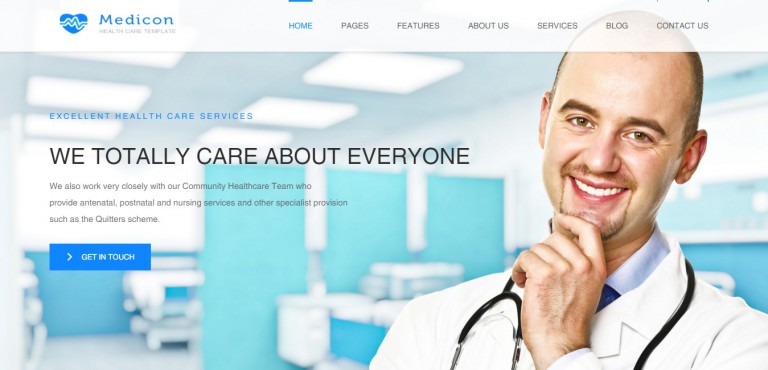This is a detailed screenshot of the MediCon healthcare website. In the bottom right corner, there is an image of a doctor. He is dressed in a white lab coat with a black stethoscope around his neck and a blue collared shirt underneath. The doctor, who appears to be balding with short hair and a goatee, is posed with his head tilted to the side and one hand up to his chin in a "thinker" style pose, while sporting a big smile. At the top of the website, within a white border, it reads "MediCon Healthcare Template" next to a blue heart logo featuring a lifeline graphic. The website menu includes the options: Home, Pages, Features, About Us, Services, Blog, and Contact Us. In the central image area, the text "Excellent Healthcare Services" is displayed, although "Health" is misspelled as "Heallth." Below this text, it states, "We totally care about everyone. We also work very closely with our community healthcare team who provide antenatal, postnatal, and nursing services and our specialist provisions such as the Quitter Scheme," accompanied by a blue button labeled "Get in Touch."